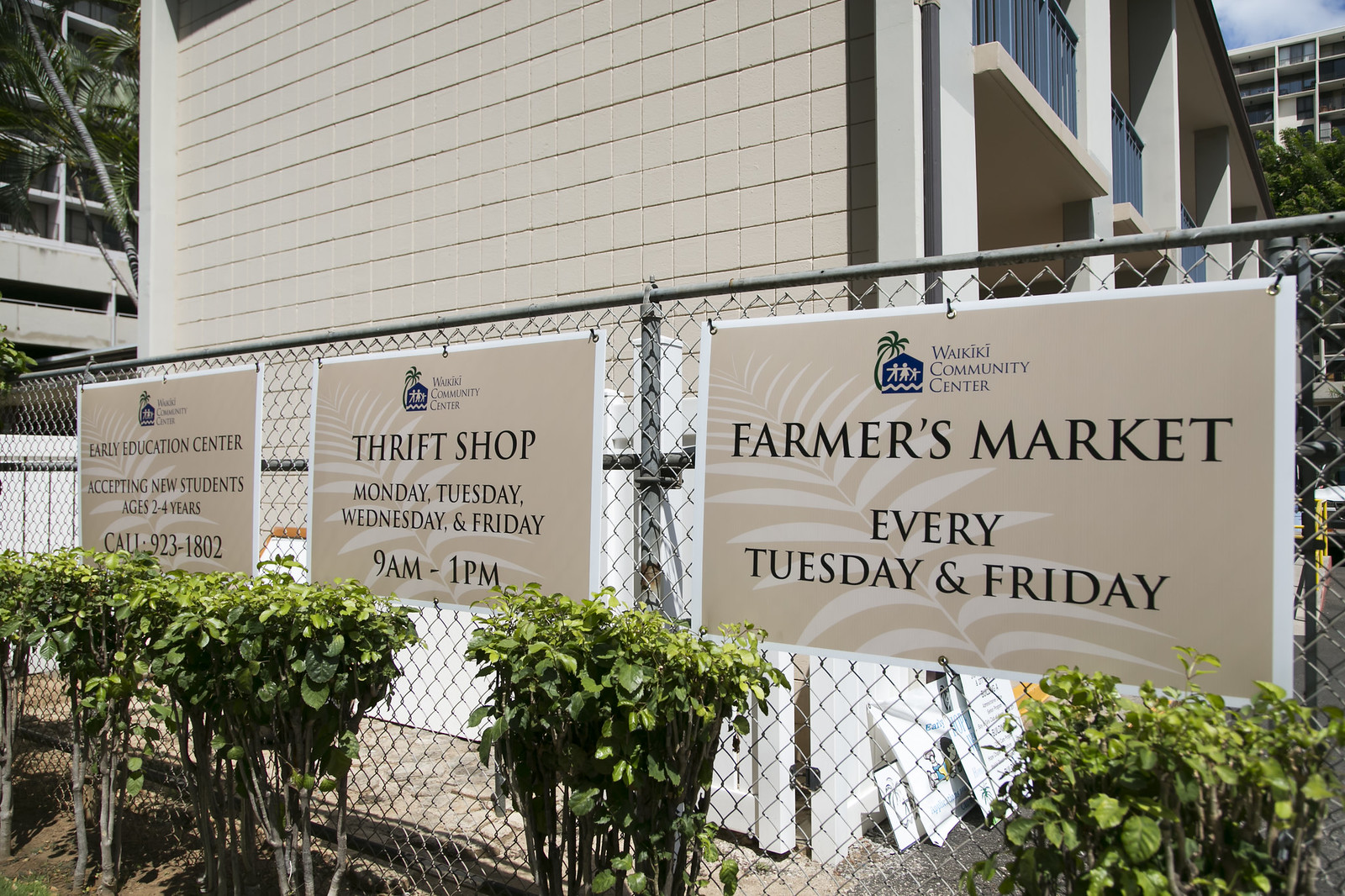In this vibrant photograph taken in a city or neighborhood on a sunny day, sunlight casts its warmth across everything, revealing a small patch of blue sky in the upper right corner. The backdrop features a mix of either office buildings or apartment buildings, characterized by their white or off-white tiled walls, possibly extending two to three floors high. Amidst the greenery, a chain-link fence stands in front of the blank facade of one such building. In the foreground are lush bushes and plants, casting shadows on the fence that holds three prominent signs. Each sign displays "Waikiki Community Center" along with a logo depicting stick figures inside a blue house shape with a palm tree. The sign on the right advertises a "Farmers Market" taking place every Tuesday and Friday. The central sign informs about a "Thrift Shop," open Monday, Tuesday, Wednesday, and Friday from 9 a.m. to 1 p.m. The leftmost sign, slightly less legible, is about the "Early Education Center" with a phone number and description beneath. All signs share a similar beige background adorned with a white palm tree leaf motif.